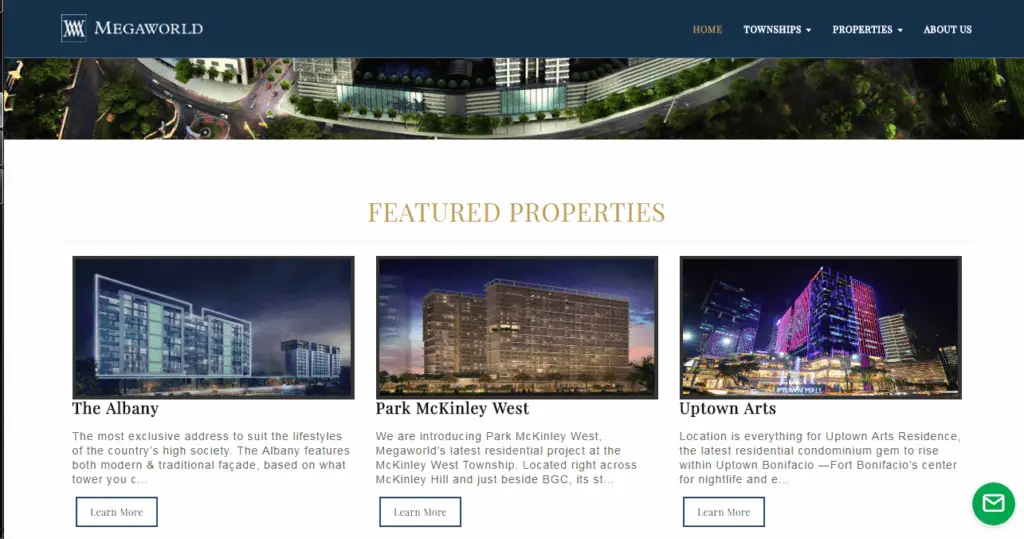In this image, we are viewing a screenshot of the Mega World website, set against a midnight blue background. Centrally displayed in bold white text is "Mega World," accompanied by a logo to its left. Positioned to the right of the text, a menu reads "Home," "Townships" with a pull-down arrow, "Properties" with a pull-down arrow, and "About Us." 

Below this menu, on a white background with gold text, the words "Featured Properties" stand out prominently. The leftmost section beneath this heading features a color photograph of a high-rise building named "The Albany." The text describes The Albany as "the most exclusive address to suit the lifestyles of the country's high society," highlighting its mix of modern and traditional façades depending on the tower. A "Learn More" button is also visible.

To the right, an image taken during the evening sunset showcases another high-rise named "Park McKinley West." The caption introduces Park McKinley West as Mega World's latest residential project located at the McKinley West Township.

Further to the right, the third property, "Uptown Arts," is mentioned. The caption underscores the importance of its location for the residents of Uptown Arts.